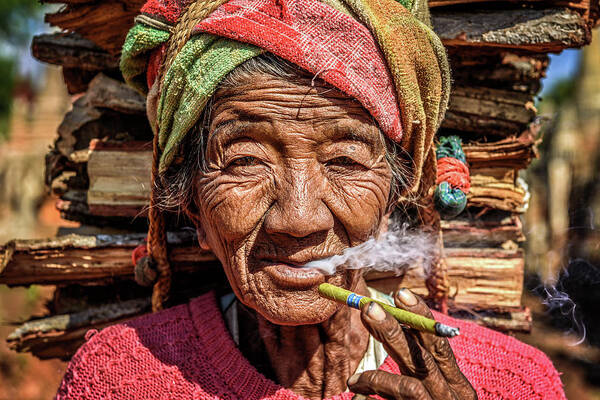This color photograph captures an elderly woman with deeply wrinkled, very dark brown skin, suggesting she has spent much of her life outdoors. She is smoking a tightly wrapped cigarette or cigarillo in bright lime-yellow paper, with smoke curling from her mouth. Her attire includes a pink cable-knit sweater and a colorful headscarf that is loosely draped over her head, featuring vibrant shades of red, green, and orange. The headscarf and sweater create a striking contrast. The woman has distinctive facial features, including a broad flat nose and slitted eyes, making her ethnicity ambiguous but possibly suggesting Asian or Indigenous heritage, perhaps from regions such as Mongolia or South America. The woman appears to be either resting against or carrying a load of chopped wood on her back, with the wood rising from her shoulders and disappearing out of the frame. Her expression conveys enjoyment, as she seems to be smiling while carrying out her daily activities under the sun.